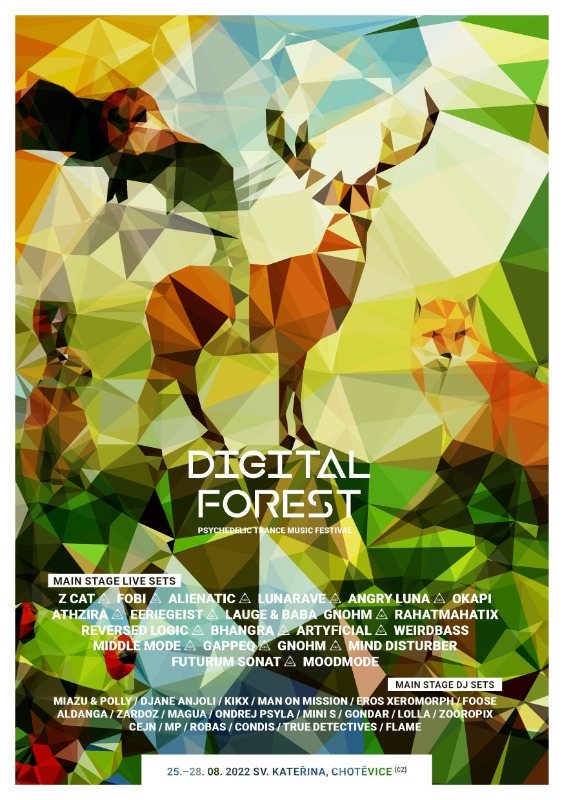The image appears to be an artistic poster for a live theater performance or an event named "Digital Forest." The design features a prismatic arrangement of multi-colored diamond and angular shapes in various shades of yellows, oranges, blues, and greens. Wildlife images are intricately interspersed through these geometric cuts, including a prominent brown and orange moose in the center, an eagle with black wings, an orange head, and a yellow beak on the top left, and potentially a lion or tiger with similar color patterns to the right. Other animals such as a deer, bobcat, owl, rabbit, fox, and frog are also depicted within these colorful, angular fragments.

Central to this intricate design, the text "Digital Forest" appears in white, flanked by greenery. Below it, the subtitle "Psychedelic Rain Dance Music Festival" is mentioned, emphasizing the event's theme. Additional information is provided near the bottom, listing performers like Z-cat, Phobia Lunatic, Lunar Rave, Angry Luna Okapi, and Ath Zebra among others, signifying "Main Stage Live Sets" and "Main Stage DJ Sets."

At the bottom of the poster, there's a white section with further details including the event date, "25-28.08.2022," and the organizer's name, "S.V. Katerina Schotterweiss."